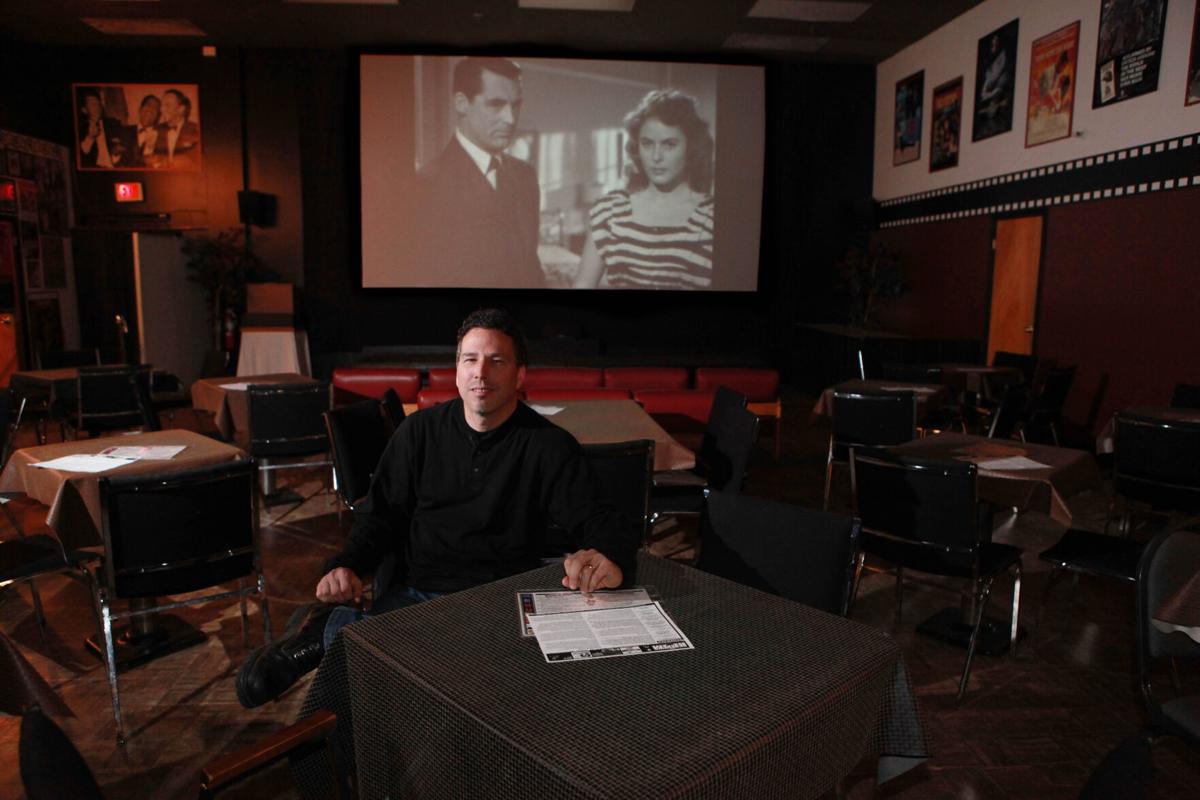In this image, a man with black hair, dressed in a black shirt, jeans, and black shoes, is seated at a table draped with a check-patterned tablecloth, working on two pieces of paper. He appears to be in a themed restaurant or small theater setting, surrounded by several similarly covered tables, many of which are empty with scattered papers. The ambiance is decorated with black-and-white movie posters, and old film reels run as a border along the walls, enhancing the retro film theme. Behind the man, a large screen displays a black-and-white movie featuring a man in a suit and a woman in a striped dress. Additional posters and photographs, including an image of men at an old movie premiere, add to the nostalgic decor. To the left of the screen, which is above a red leather couch, an exit sign is visible beneath another old-time poster.